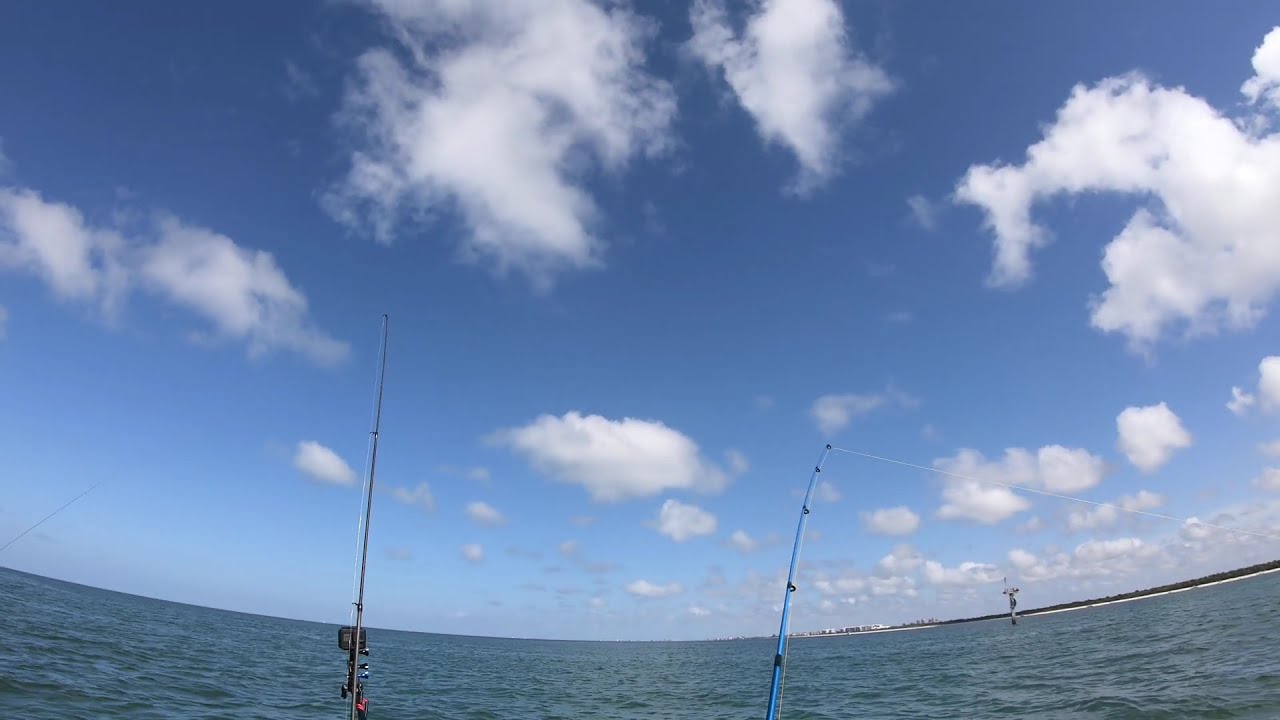The image captures a serene fishing scene, likely taken from a small boat suggested by the camera's fisheye lens effect, reminiscent of a GoPro camera's view. The focal point is two fishing poles: a black one on the left and a light blue one on the right, both with their lines cast into the water, awaiting a catch. The backdrop is a large body of water, possibly an ocean or a vast lake, bordered by a distant, almost indistinct cityscape or coastal line with a hint of buildings or houses. The sky above is a mix of blue with scattered white clouds, giving the scene a mild, somewhat cloudy ambiance. The overall lighting implies it's later in the afternoon, around 3 or 4 p.m., as the daylight begins to wane. There are no visible people in the shot, but a few distant boats can be perceived, adding to the tranquil atmosphere.